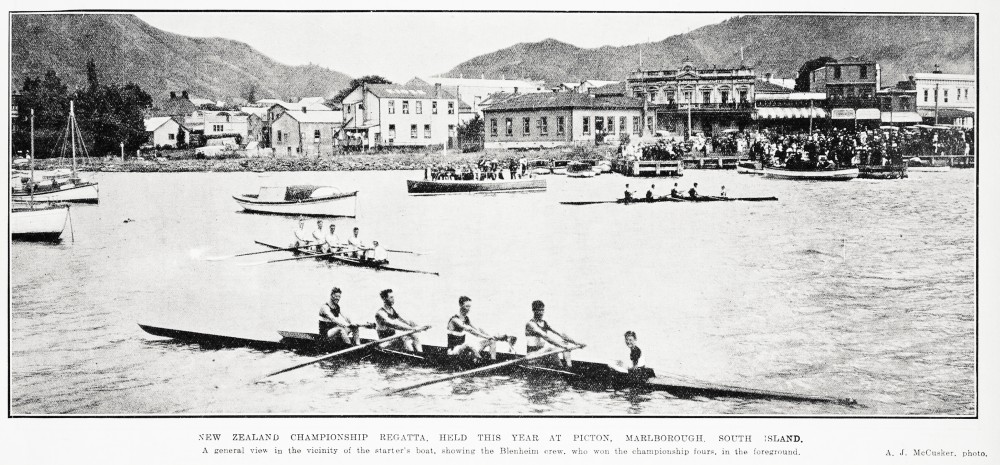This rectangular, black-and-white photograph, wider than it is tall, captures a historic moment from the New England Championship Regatta, held this year at Picton, Marlborough, South Island. The image, attributed to AJ McConquer, shows a general view in the vicinity of the starter’s boat, with the victorious Blenheim crew in the foreground. The scene is set on a body of water, framed by mountains and a village with numerous buildings and trees along the shoreline.

In the foreground, three long boats, each manned by five men—four rowers and one coxswain—are visible. Clad in tank tops and shorts, the men are holding their oars, suggesting a moment either just before or after the race. The boats are aligned, seemingly in a ready or resting position. The far background features a clear sky above the mountainous terrain and village, providing a picturesque yet nostalgic backdrop typical of regatta events from many decades past. Spectators line the riverbank, adding a human element to the serene and competitive atmosphere of the regatta.